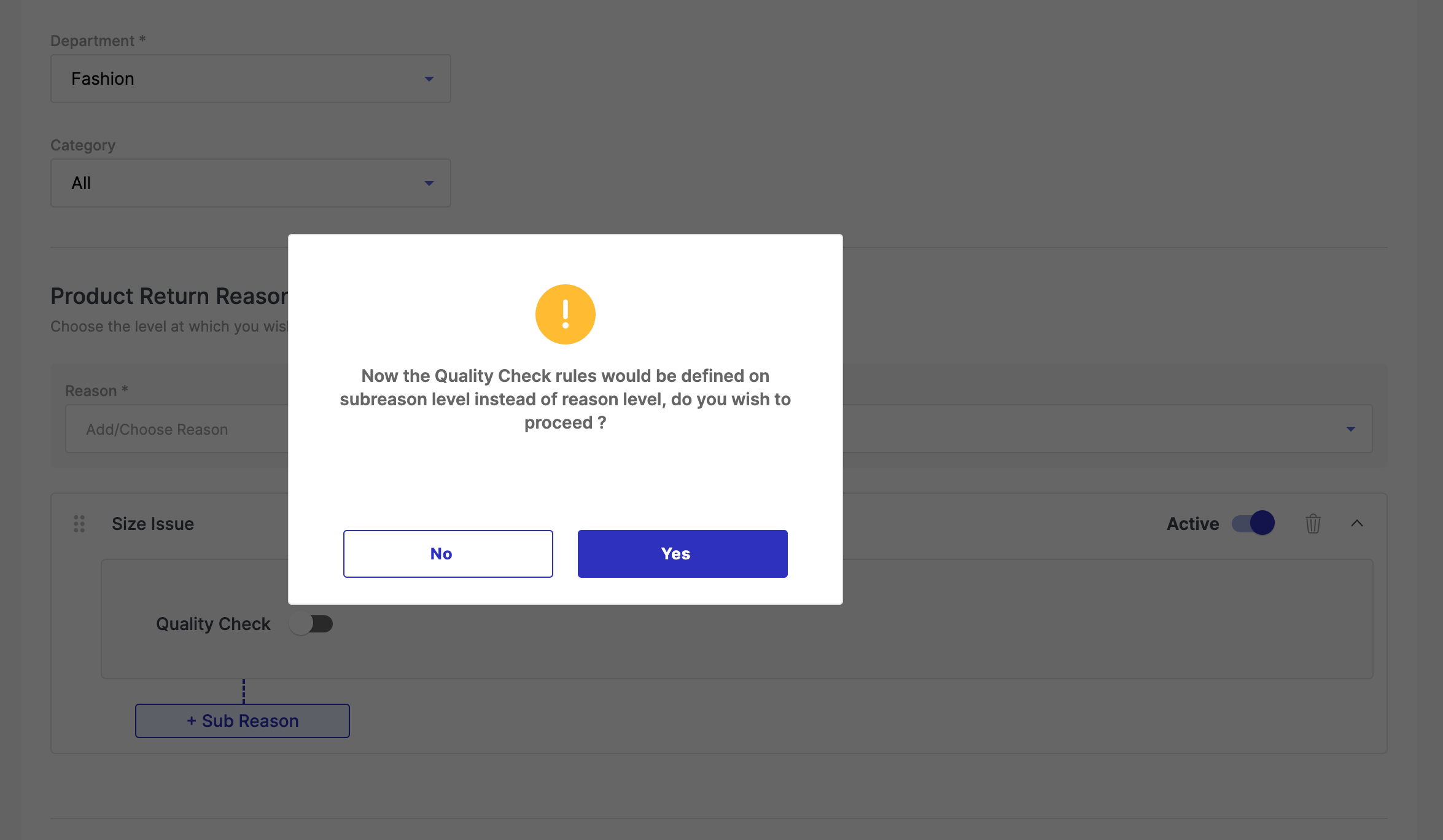In the image, we see a user interface with a grey background. Central to the image is a prominent white square pop-up. At the top of this pop-up, there's a yellow-orangeish circle containing a white exclamation point. Below the circle, the text reads: "Now the quality check rules would be defined on sub-reason level instead of reason level. Do you wish to proceed?" There are two buttons beneath this text – a white "No" button with blue text and a blue "Yes" button with white text.

On the left side of the screen, details are listed in a structured format. At the top, there is a "Category Department" section labeled "Fashion Category" with the option "All" indicated. Below, under "Product Return Reason," there is a "Reason" field that can be filled out. Continuing down, a "Size Issue" section is mentioned. Below this is a "Quality Check" option which is toggled off. Further down, "Sub-reason" is highlighted in blue, accompanied by an "Active" option to the right, which is toggled on with a blue button slid to the right.